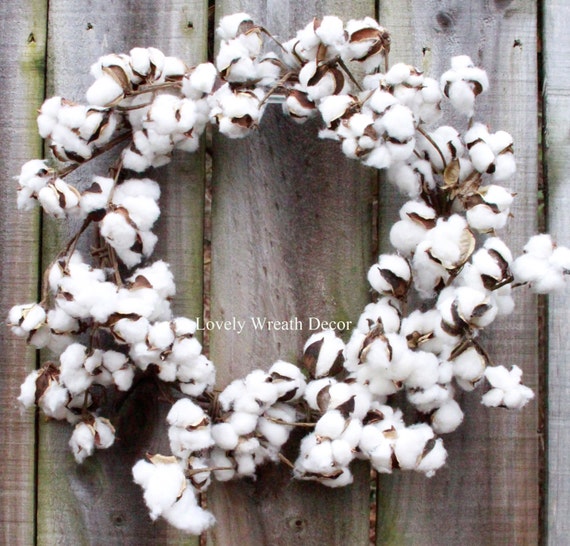A detailed image of a decorative wreath held up against a wooden slat fence. The wreath is fashioned from brown vines meticulously intertwined to form a perfect circle. At the bottom center of the wreath, delicate white cotton puffs are arranged to resemble flower tips, creating a lovely contrast against the earthy tones. Surrounding these cotton puffs are an array of brown leaves, which add to the natural and rustic charm of the decor. The backdrop of the image features a wooden slat fence, composed of vertical boards placed side by side. The fence exhibits a light brown and light gray gradient, with streaks of darker wood grain running throughout, offering a subtle yet appealing background that enhances the overall composition of the wreath.